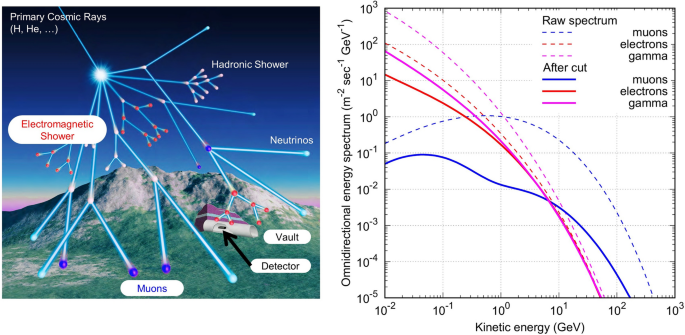The image features a detailed infographic on cosmic rays. On the left side, there is an illustration of a mountain range with labels such as "primary cosmic rays" and specific elements like "H for hydrogen" and "He for helium." A visual depiction shows a single cosmic ray beam striking a point, resulting in a branching tree-like structure of various secondary particles, forming an "electromagnetic shower" that breaks into hadronic showers, neutrinos, and muons. Additionally, there are labels for a "vault" and a "detector" located at the bottom of the mountain illustration.

The right side of the image includes a graph plotting 'kinetic energy' on the horizontal axis, ranging from 10^-2 to 10^3, against the 'omnidirectional energy spectrum' on the vertical axis, spanning from 10^-5 to 10^3. This graph displays curved lines that differentiate between raw spectra and aftercut spectra of muons, electrons, and gamma rays, culminating in a comprehensive view of the energy distribution of particles resulting from cosmic radiation entering Earth's atmosphere.